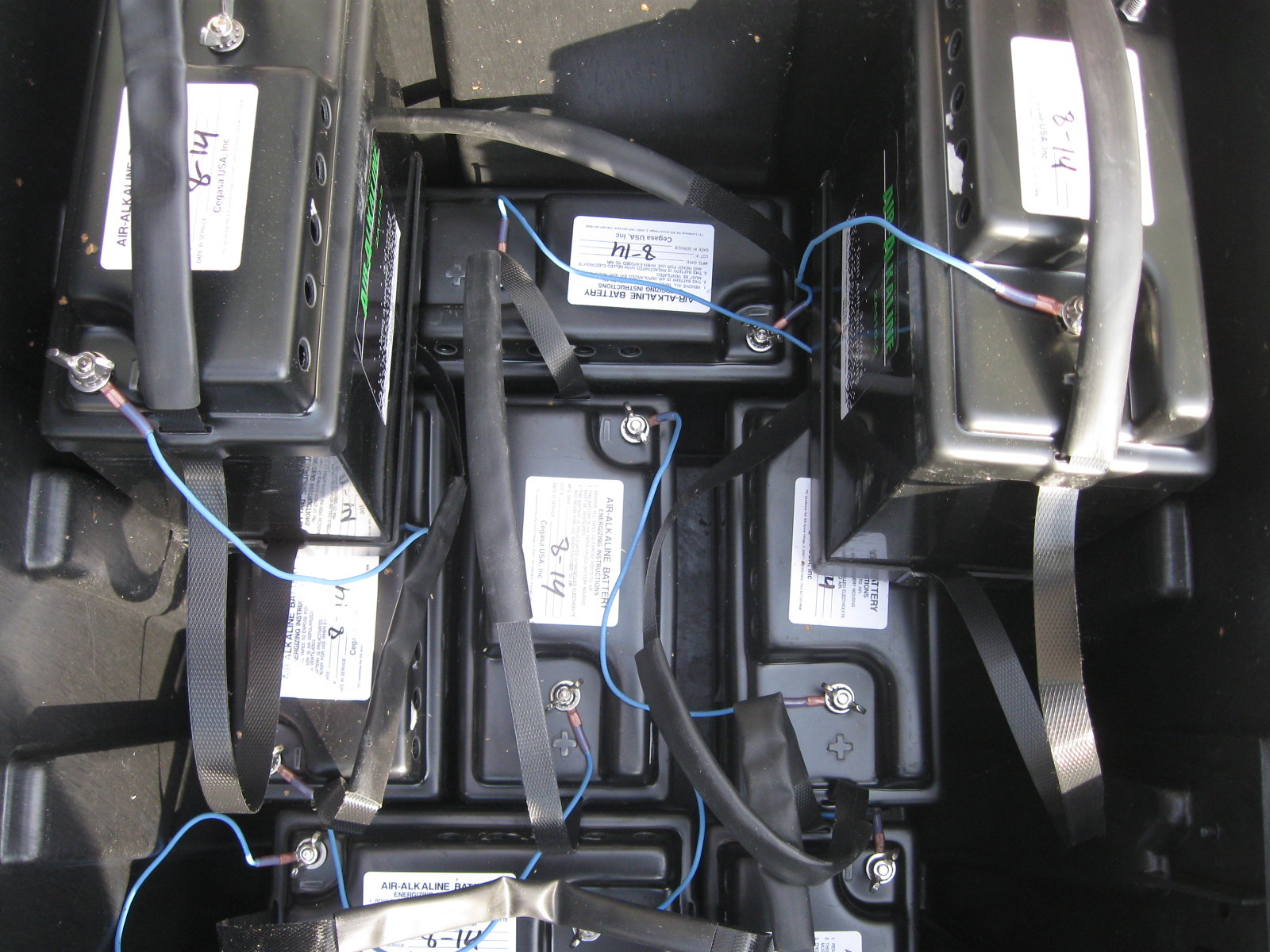The photograph features a group of large, black batteries commonly used in vehicles such as cars, RVs, boats, or golf carts. Seen from above, the image captures at least eight batteries arranged in a mix of horizontal and vertical positions, though there could be more just out of frame. Each battery is topped with a closed plastic cover, from which labeled positive and negative terminals protrude. The batteries are interconnected with blue leads, which are secured with wing nuts. All the batteries display a white rectangular sticker with the handwritten date "8-14" and the word "alkaline." The background of the photograph remains dark, highlighting the arrangement and connections of the batteries. Some batteries show signs of being wired in series, with leads running from the negative terminal of one to the positive terminal of another.